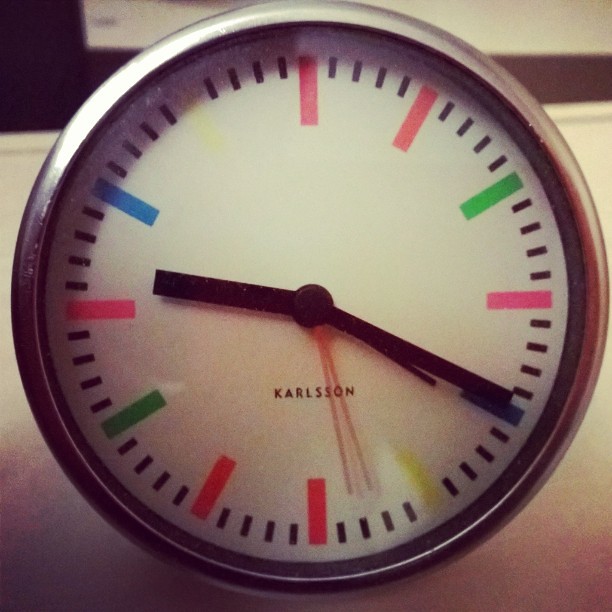This image showcases a close-up view of a stylish Karlsson (spelled K-A-R-L-S-S-O-N) clock, emphasizing its modern design elements. The round clock features a sleek stainless steel case that frames its pristine white face. Instead of traditional numbers, the clock displays vivid, bold lines in various colors such as green, pink, yellow, red, and blue to mark the hours. Black lines denote the minutes in between. The clock has distinctive bold black hour and minute hands, with the minute hand being an especially thin, pale pink needle, adding a subtle touch of elegance. The clock appears to be resting on a white table, evident from the shadow cast beneath it, though its precise mounting (wall or table) is ambiguous. The clarity in design and the use of vibrant and contrasting colors make this timepiece a striking centerpiece.